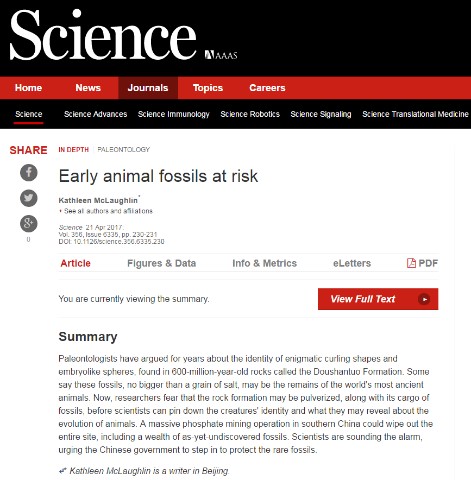This screenshot captures a webpage from an unidentified science-focused platform. The webpage's name or platform’s identification is not visible. Dominating the top of the screen is a thick black bar with the word "Science" prominently displayed. Beneath this, a red navigation bar features five tabs labeled Home, News, Journals, Topics, and Careers. The Journals tab is currently selected, revealing a dropdown menu listing different sections: Science, Science Advances, Science Technology, Science Robotics, Science Signaling, and Science Transformations. The main content highlights an article titled "Early Animal Fossils at Risk," accompanied by a brief summary. A red button beneath the summary invites users to view the full text of the article.